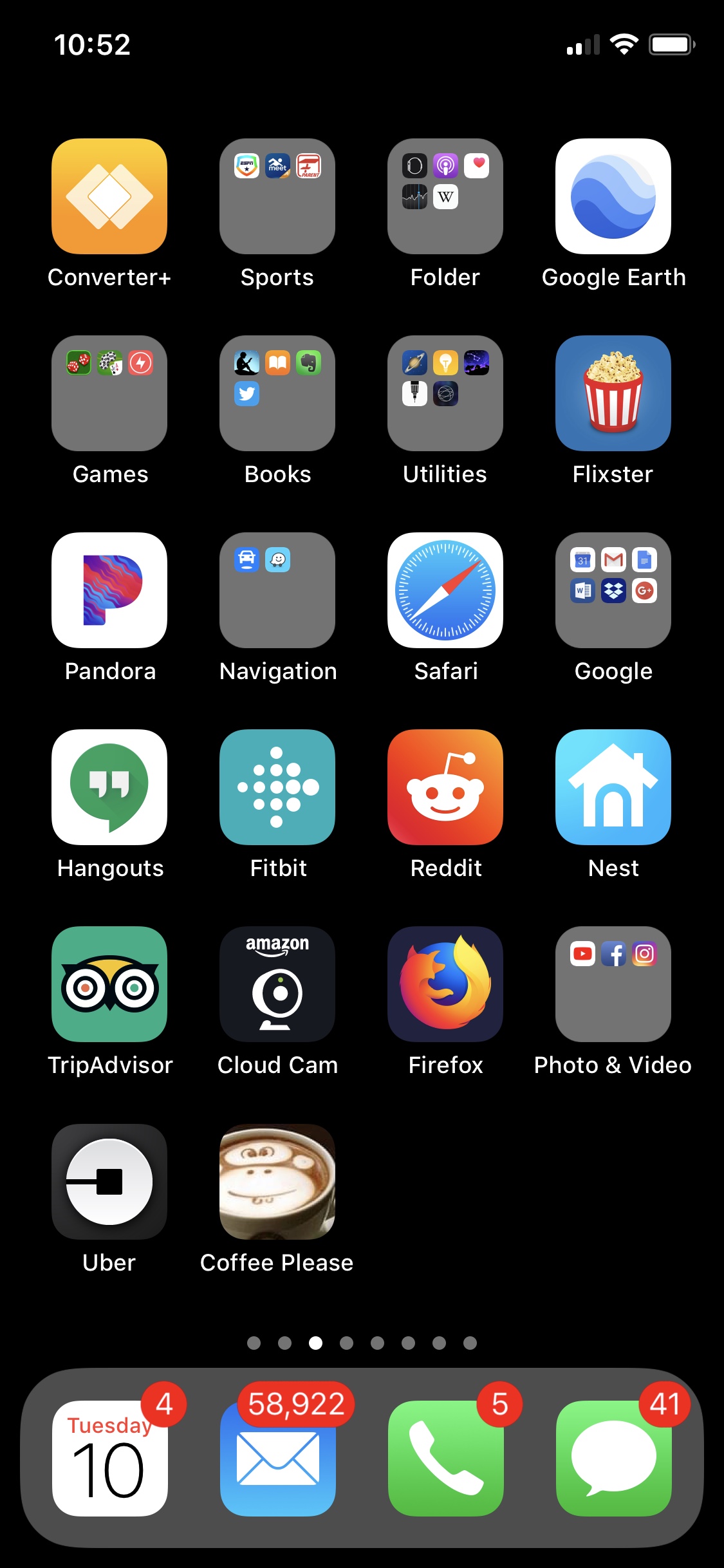This is a meticulously detailed screenshot of an iPhone home screen. The background features a black wallpaper, providing a stark contrast to the app icons. At the bottom, the dock displays four essential apps: Calendar (with 4 notifications), Mail (overwhelmed with 58,922 notifications), Phone (with 5 notifications), and Messages (with 41 notifications). 

The time displayed at the top of the screen is 10:52, and the device shows a strong Wi-Fi connection and a nearly full battery. The top row of apps includes icons for TripAdvisor, Firefox, Reddit, an app labeled "Next," and a folder named "Google." Also present on the screen are the Safari browser, Pandora, and Flixster apps. 

The user has organized their apps into several folders: "Sports," "Folder," "Games" (with three apps), "Books" (with four apps), "Utilities" (with five apps), and "Navigation" (with two apps). Additionally, the Fitbit app indicates that the user likely owns a Fitbit device. This screenshot encapsulates an iPhone user's well-organized but heavily notified home screen.